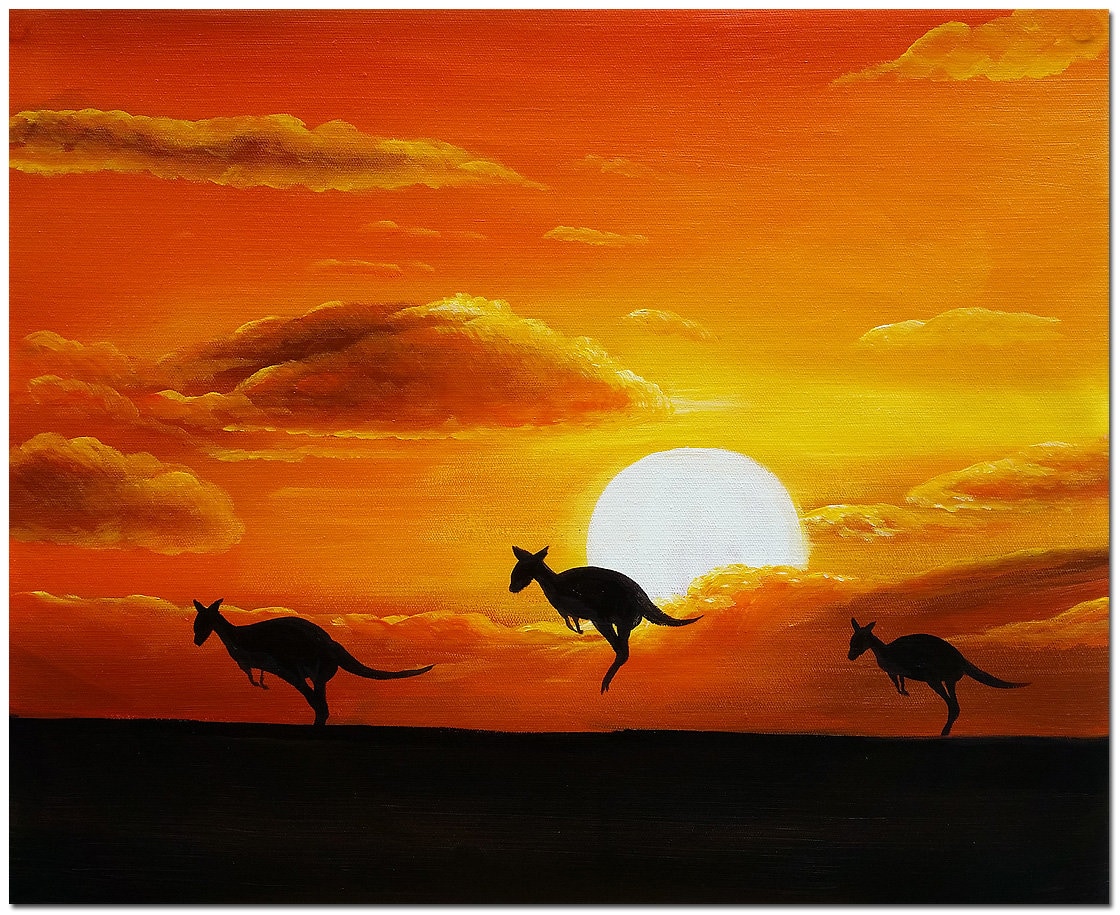This image captures a stunning, minimalist painting of an outdoor scene featuring a vibrant and dynamic sunset. The upper three-quarters of the canvas are dominated by a rich, deep orange sky with variations throughout, transitioning to yellows in the vicinity of a bright, round Sun emerging from a patch of lighter, almost white-yellow clouds. The bottom quarter of the painting represents the ground, rendered in stark black, providing a striking contrast to the vivid sky above. Silhouetted against this glowing backdrop are three kangaroos, each in a different stage of movement: one with its back feet on the ground, poised in the foreground; another mid-jump, leaping in front of the radiant Sun at the center; and a smaller kangaroo with its back feet just touching the ground. The overall effect is both dynamic and serene, capturing the essence of the natural landscape at dusk.